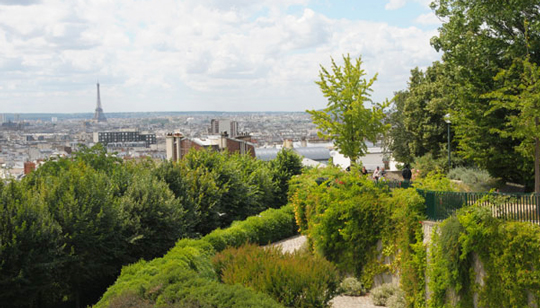This is a detailed daytime photo capturing a panoramic view of Paris from a hillside park above the city limits. In the foreground, there is a path bordered by a short, three-foot-tall green metal fence on the right side. Beyond the fence, a group of people can be seen walking in the distance. The area is lush with green trees, bushes, and plants, giving it the appearance of a garden or national park. On the left side, trees cascade down the hillside, framing the cityscape below. The vast cityscape of Paris stretches out flat towards the horizon, dominated in the background by the iconic Eiffel Tower rising prominently above the dense collection of buildings. The sky overhead is filled with billowing white clouds, casting a soft, overcast light across the scene, making it a calm, shady day. The overall view beautifully captures the juxtaposition of natural and urban landscapes.